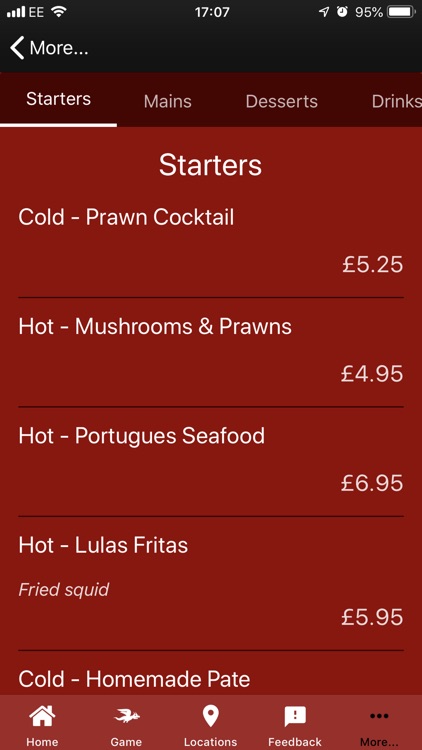The image displayed on the phone screen shows a menu interface for a restaurant. The phone's time is 17:07 and the battery is at 95%. The menu is categorized into sections: Starters, Mains, Desserts, and Drinks, with an arrow on the left for navigation to more options. The background colors transition from black to maroon and then to a reddish hue. 

At the top of the screen, the word 'Starters' is prominently underlined and displayed in large letters. The first item listed is a Cold Prawn Cocktail priced at $5.25. Following this is a dish of Hot Mushrooms and Prawns costing $4.95, then a Portuguese Seafood option priced at $6.75. There is also an offering of Hot Lulas Fritas, identified as fried squid, which costs $5.95. Additionally, there is a mention of a Cold Homemade Plate, though the description is vague, suggesting the need to scroll further to see details.

At the bottom of the screen, typical navigation icons are present: Home, a bird icon labeled 'Game', Locations, Feedback, and a 'More' option represented in black with three lines.